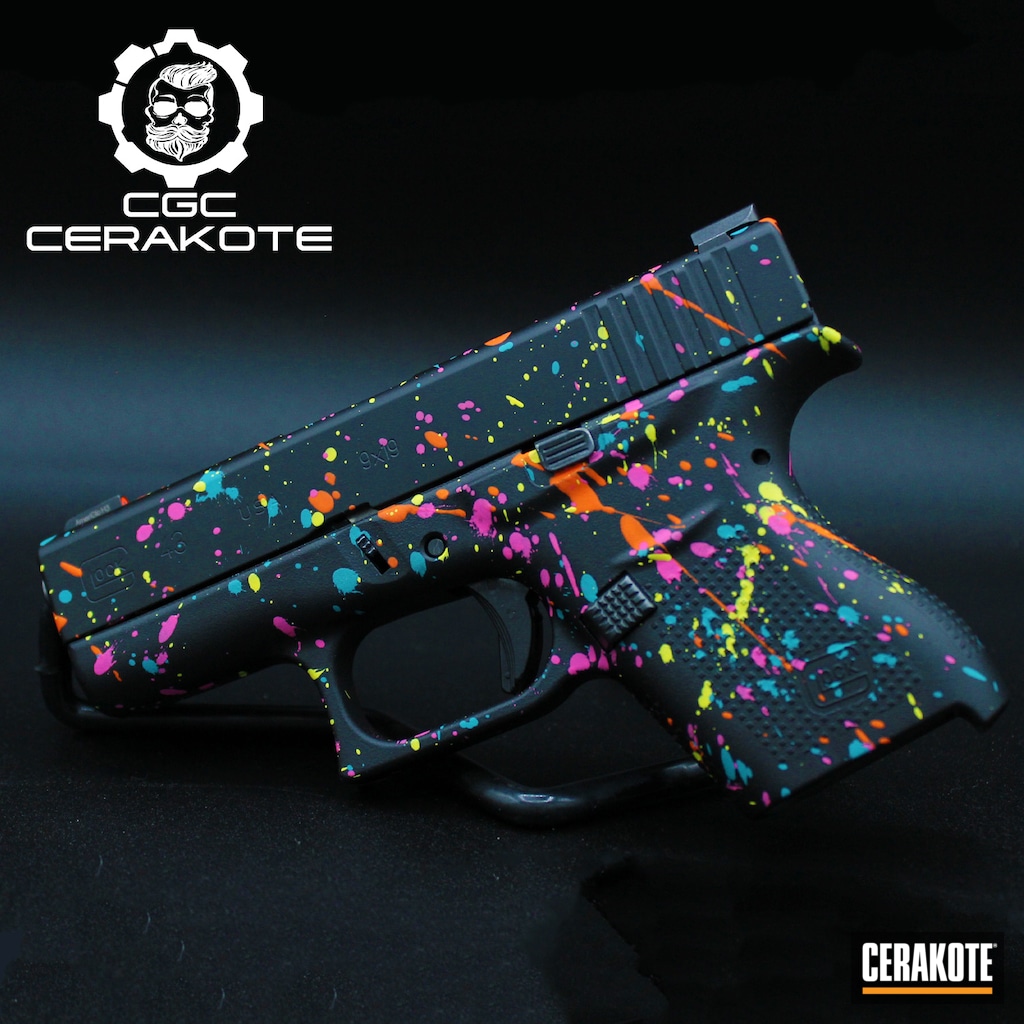This photograph features a black handgun, likely a Glock, prominently showcased against a dark gradient background. The handgun is uniquely decorated with an irregular multicolored paint splatter design, featuring vibrant streaks and speckles of blue, yellow, red, magenta, pink, orange, and teal. In the upper left corner of the image, the logo and name "GCGC Cerakote" appear, accompanied by an icon of a gear with a bearded man's face. In the bottom right corner, the word "Cerakote" is displayed in white font with an orange underline. This image appears to be an advertisement for a specially designed Cerakote handgun, emphasizing its custom, artistic paint finish.